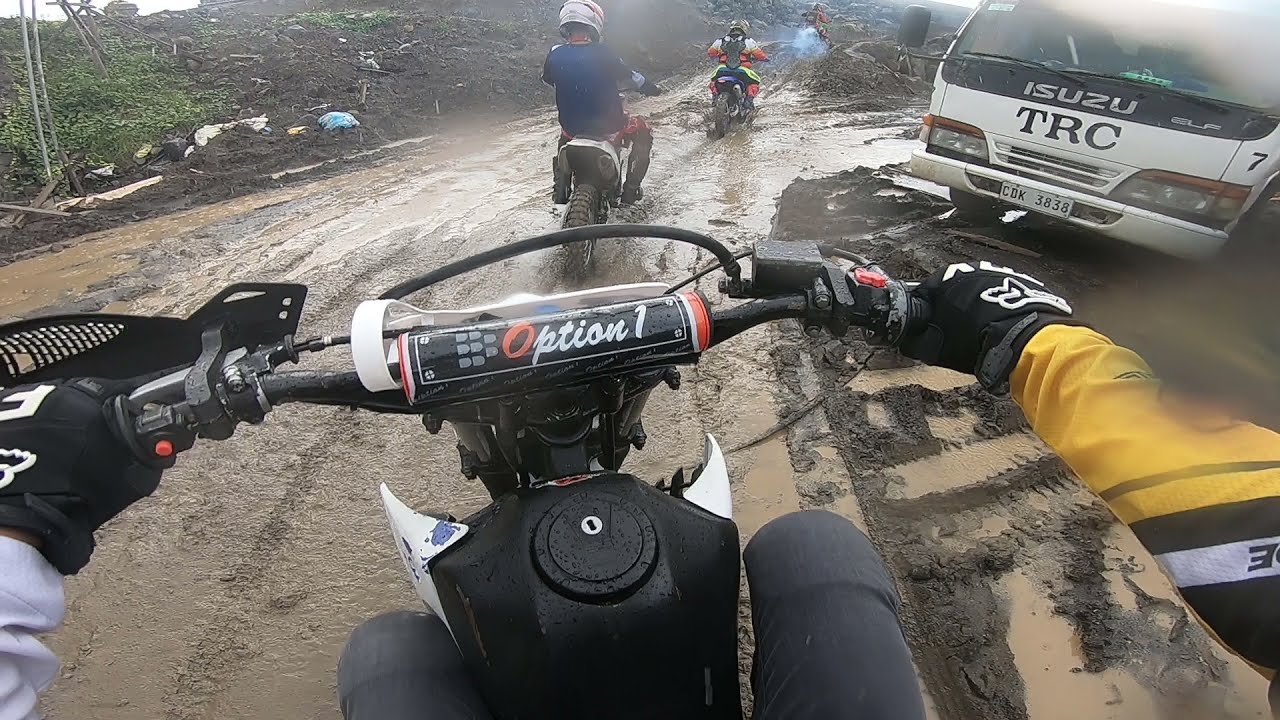The photograph captures a helmet camera view of a dirt bike rider navigating a muddy dirt track. The rider wears a distinctive outfit with a bright yellow sleeve with black accents on the right arm, a white sleeve on the left arm, black gloves, and black pants. Prominently displayed in the center of the handlebars is a decal reading "Option 1," with the letters in a cursive font and an orange-red "O."

Ahead on the muddy and wet path are three other bikers: one in a blue shirt with a white helmet, another in an orange suit with a dark helmet, and the third biker's details are less distinct. The trail is dotted with pools of dirty, muddy-brown water. To the right, a white truck with the markings "Isuzu TRC" and a European license plate "CDK3838" faces the camera. On the left side of the image, patches of green grass and churned-up black soil and mud are visible. The scene is brightly lit, indicating that the photo was taken during the daytime in natural light.